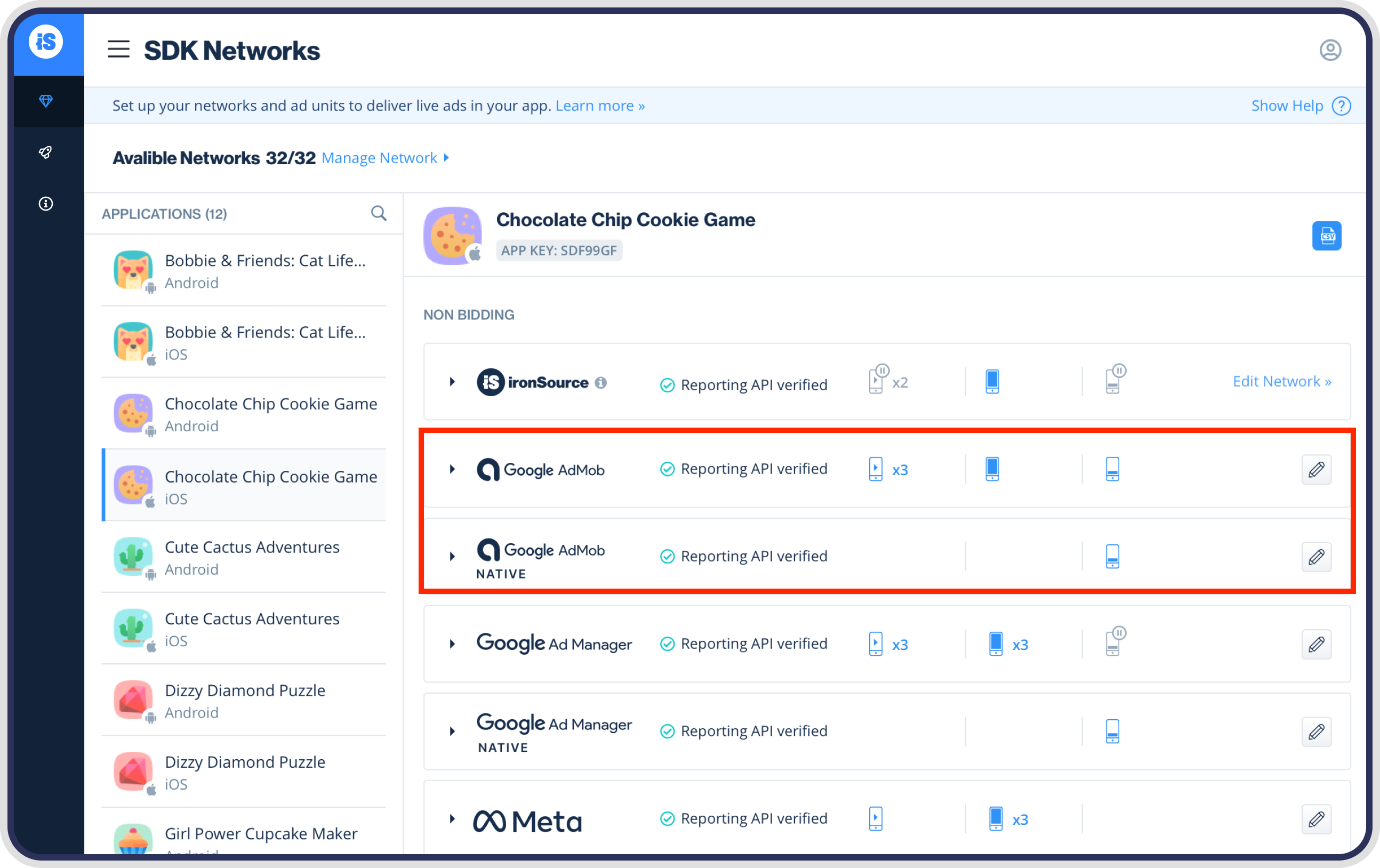This is a horizontal digital interface displayed within a framed window on a computer or smart device. The interface is encased in a light gray border with an outer black border featuring rounded edges, set against a white background.

On the far left, there is a vertical blue sidebar containing a circular icon with the letters "I" and "S" inside. Below this icon, there are several clickable vertical icons. Adjacent to this sidebar is a rectangular white search box that extends horizontally. This box includes a three horizontal-line menu button for additional options and a bold label that reads "SDK Networks." On the far right of this bar is a clickable profile picture icon, which users can interact with to access their profile options.

Beneath this section, a light blue strip runs across the interface, featuring the text: "Set up your networks and add units to deliver live ads in your apartment." Towards the right of this strip, there are two clickable options: "Learn More" highlighted in blue, and "Show Help" accompanied by a question mark icon.

Further down, a section titled "Available Networks" appears, indicating 32 out of 32 networks in black font, and a blue button labeled "Manage Networks." Below this, a search functionality is indicated by a magnifying glass icon next to a text box labeled "Applications". It indicates there are 12 applications, each listed with their icon, name, and platform (either Android or iOS).

The highlighted application in this list is "Chocolate Chip Cookie Game," shown with its icon and status "Now Bidding." Under this application, specific sources such as "IronSource," "Google AdMob," and "Google AdMob Native" are listed, each accompanied by a red-bordered box containing various icons and verification stamps such as "Reporting API Verified."

The interface continues to list different options and applications in a detailed and structured manner as the user scrolls down.